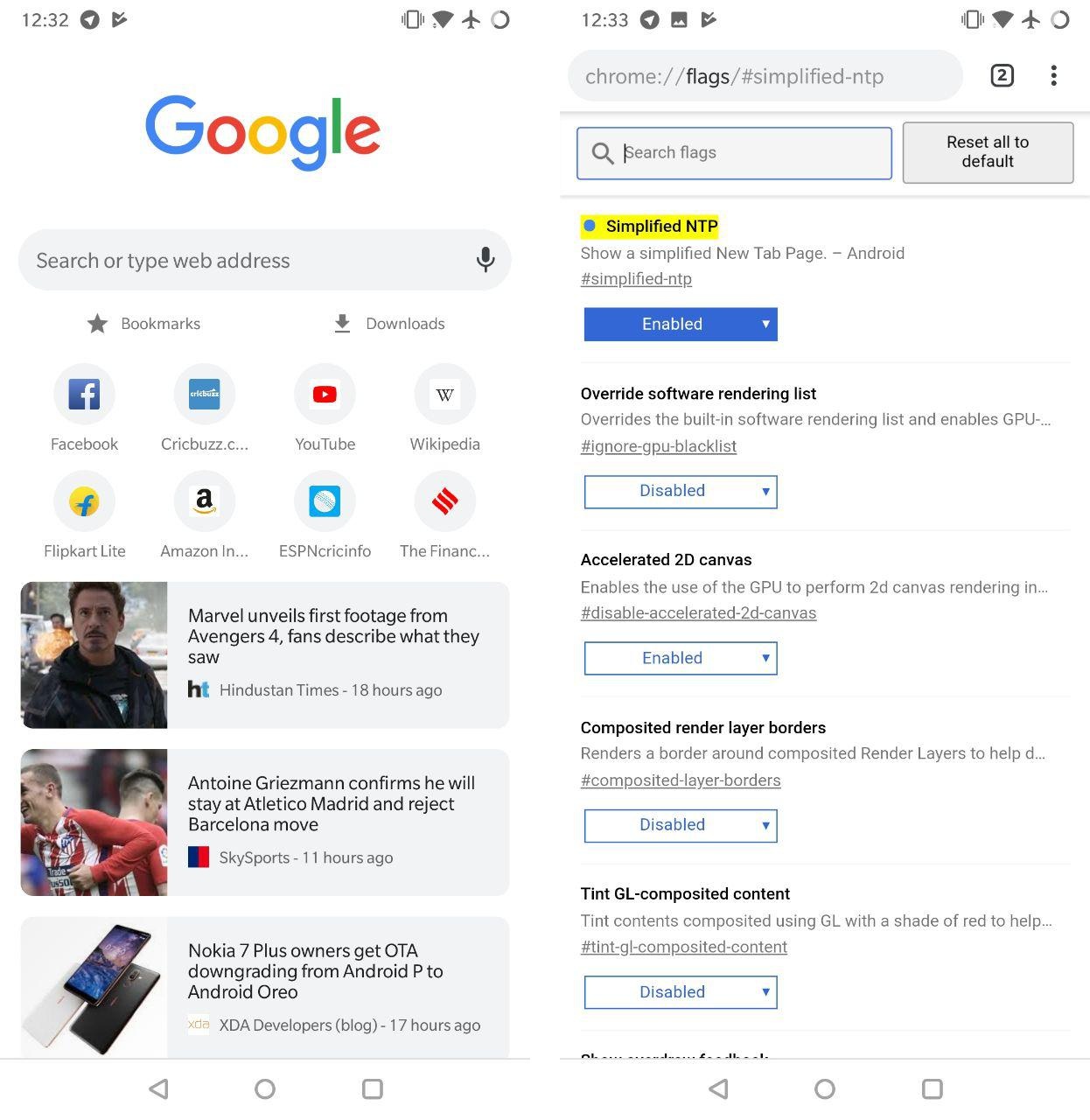This image showcases two mobile phone screens side by side with a clean, white background. The top of both screens prominently displays the time "12:32." Adjacent to the time are several icons: a circular arrow, a triangle with a check mark, signal bars indicating airplane mode, Wi-Fi status, a vibrate symbol, and a circular icon suggesting a download in progress.

The right screen is more detailed, featuring the Google logo in its iconic blue, red, yellow, and green colors. Beneath the logo lies a search bar labeled "Search or type web address." Further down, there are categories labeled "Bookmarks" and "Downloads," followed by various app icons including Facebook, Circa News, BuzzFeed, YouTube, Wikipedia, Flipkart, Flipkart Lite, Amazon India, ESPN, and The Financial Times.

Below these icons, the screen displays three news items, each accompanied by a photograph:
1. "Marvel unveils first footage from Avengers 4. Fans described what they saw." - Hindustan Times, 18 hours ago.
2. "Antoine Griezmann confirms he will stay at Atletico Madrid and reject Barcelona's move." - Sky Sports, 11 hours ago.
3. "Nokia 7 Plus owners get OTA downgrade."